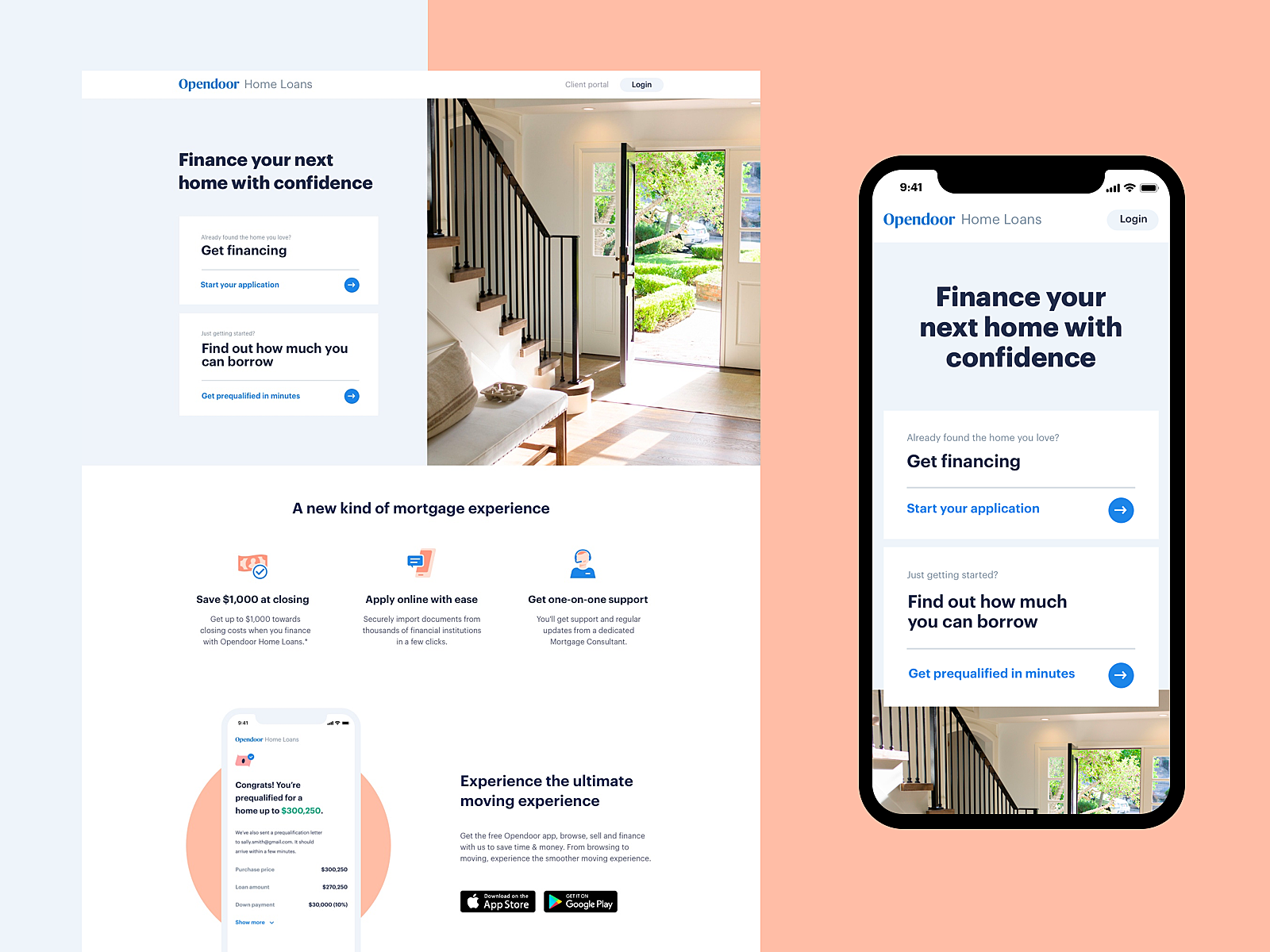The screenshot captures a promotional message displayed on a smartphone screen, divided into three sections. The first section features a message encouraging users to "Finance your next home with confidence" and provides actionable options such as "Get financing" and "Find out how much you can buy."

The second section elaborates on the mortgage experience by highlighting three key benefits: saving dollars at closing, applying online with ease, and using a mobile app available on the phone. A small icon of a phone emphasizes the app's accessibility.

The third section reiterates the call to "Finance your next home with confidence" and incorporates a visual element—a feedback wheel—accompanied by a background showing stairways, evoking the image of ascending towards new home ownership.

In essence, the screenshot is designed to guide users through a seamless and reassuring home financing process via their mobile devices.